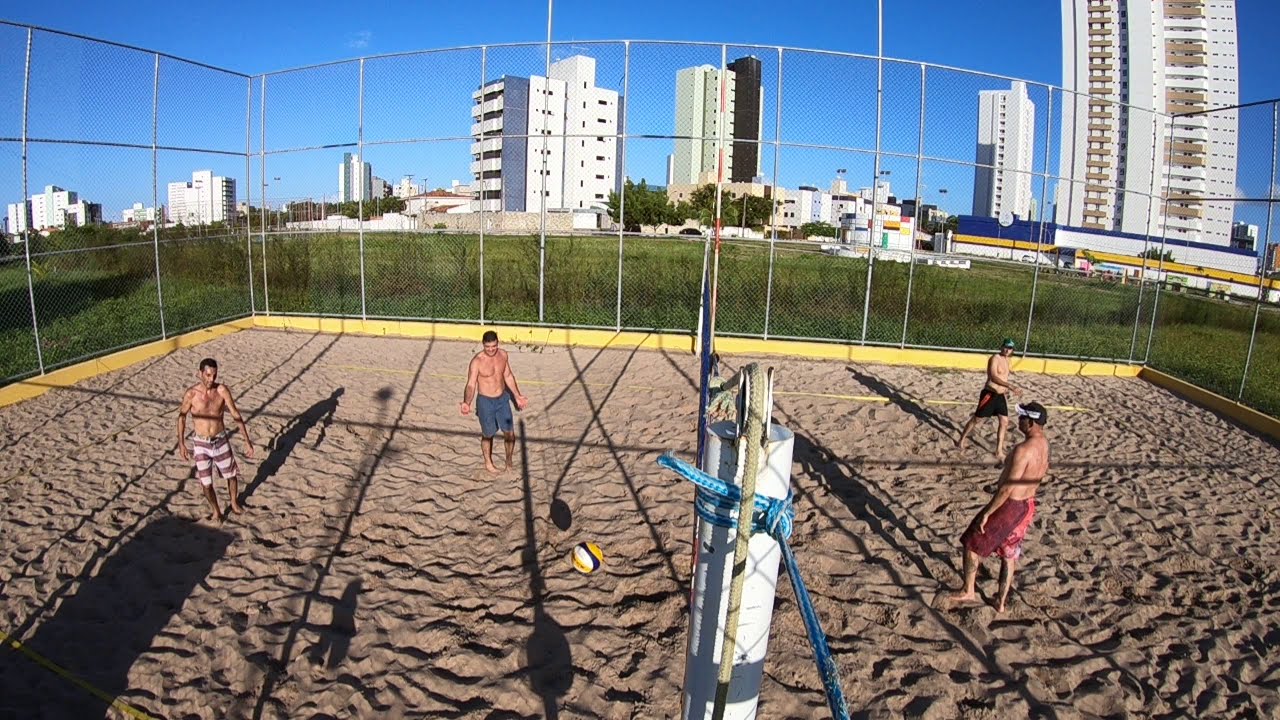In the photograph taken on a bright, clear day with a flawless blue sky, four men are playing volleyball within a large cage-like enclosure with wire fencing about 12 feet high. The scene appears to be viewed from a referee's perspective, positioned center behind the net, which divides the court evenly. Each player is clad in swimming trunks or board shorts of varying colors, and all are shirtless. The sandy ground of the court suggests a beach setting, although the wire fencing gives it an appearance reminiscent of a tennis court repurposed for sand volleyball.

On the right side of the net, one player sports a visor while another wears a hat, both engaged in active play. The opposite side mirrors this dynamic energy with two other players, one in brown-striped shorts and the other in blue shorts. The volleyball engaged in the game is mid-air, vividly colored in yellow, black, and white.

Surrounding the enclosure is a grassy field that transitions into a cityscape featuring very tall buildings and skyscrapers, visible in the backdrop. There are also some bushes and the overall environment is bathed in sunlight under the cloudless sky.